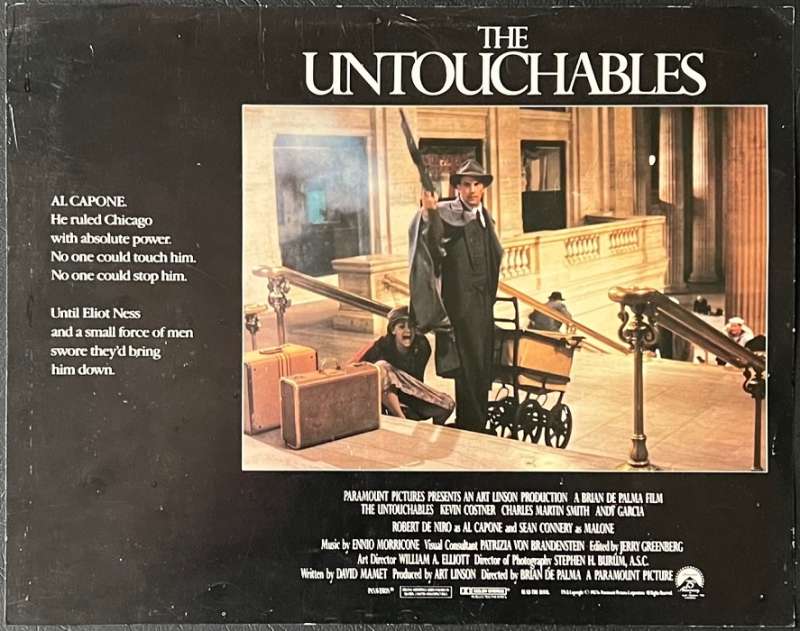This is a detailed movie poster for "The Untouchables" set against a black background with prominent white text. Centered at the top, the title "The Untouchables" stands out in large font. The left side features a quote: "Al Capone. He ruled Chicago with absolute power. No one could touch him. No one could stop him. Until Eliot Ness and a small force of men swore they'd bring him down."

The central image captures a dramatic scene: a man in a black suit, gray overcoat, and top hat, brandishes a shotgun with his right hand while holding onto a baby carriage going downstairs with his left. He's surrounded by tan steps, suggesting a grand setting, possibly a bank or public building, with white columns in the background. Next to him, a woman in a black jacket and light purple skirt appears distressed and is potentially either screaming or crying, sitting beside two pieces of luggage—one orange, one brown—at the foot of the stairs. The overall imagery evokes a sense of urgency and tension. The bottom of the poster includes credits: "Paramount Pictures Presents an Art Agent Production, a Brian De Palma Film, The Untouchables," followed by the names Kevin Costner, Charles Morton Smith, Andy Garcia, Robert De Niro as Al Capone, and Sean Connery as Malone, displayed alongside the Paramount emblem featuring a mountain and stars.